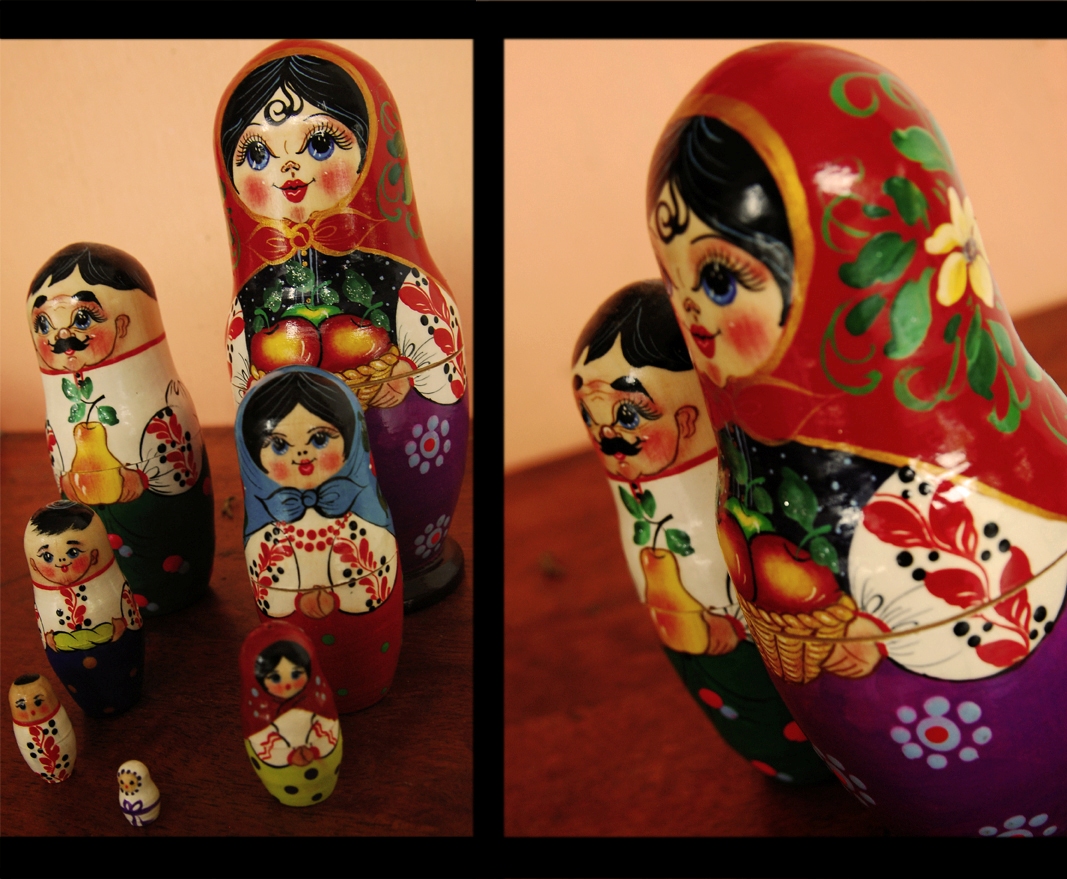This image showcases a group of Russian matryoshka (nesting) dolls, intricately painted and nested to form a detailed collection. The photograph is divided by a black line down the center. On the right side, it features the two primary nesting dolls: a taller one with a red top, a white face, apples depicted in the middle, and a purple bottom, representing a woman, and a shorter one with a male face in the center holding a pear. The left side of the photograph reveals a more extensive set, expanding on the two principal dolls by displaying their smaller nested forms. This side shows a total of seven dolls, starting with the larger woman holding a basket of apples, followed by the man holding a pear. Progressing downward in size, there is a woman with a blue head wrap and folded hands, a child or man holding a loaf of bread, a female child with a red headscarf, a male child in a white outfit, and finally, a tiny baby dressed in a white outfit with purple ribbons. These vibrant dolls, painted in hues including red, blue, gold, green, purple, white, black, tan, and green, rest atop a wooden surface against a light-colored wall backdrop. The photo captures the glossy, colorful detail of the matryoshka dolls, emphasizing their traditional ovoid shapes.